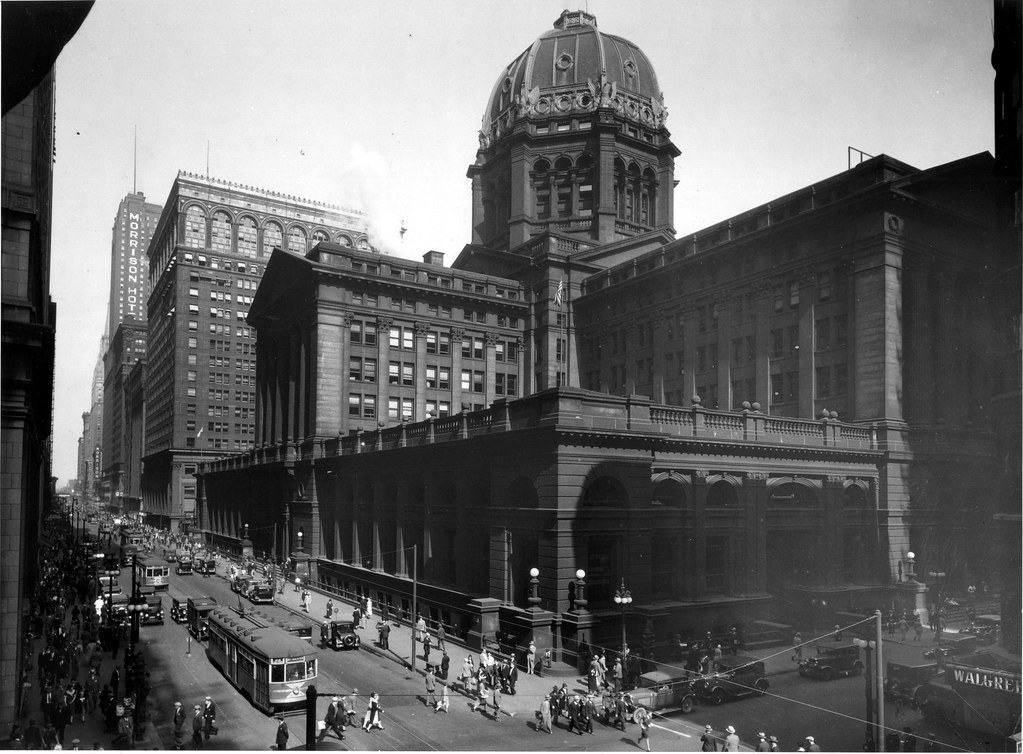This black-and-white photograph, likely from the early 1900s, captures a bustling scene in a major American city. The streets are lined with early Ford vehicles and a mix of vintage cars from possibly the 1920s to the 1940s. The sidewalk teems with people dressed in business casual attire characteristic of the era. At the forefront of the image is a large building with a distinct circular, domed top, adding a unique architectural element to the scene. The buildings along the street, constructed with brick masonry and abundant windows, exemplify early 20th-century architectural styles. Notably, a sign for the "Morrison Hotel" is visible, alongside the familiar logo of a Walgreens in the bottom right corner, cementing the urban setting. This street scene is further animated by the presence of old trolley cars and numerous street lights, painting a vibrant picture of a day in the life of a busy city during this historical period.